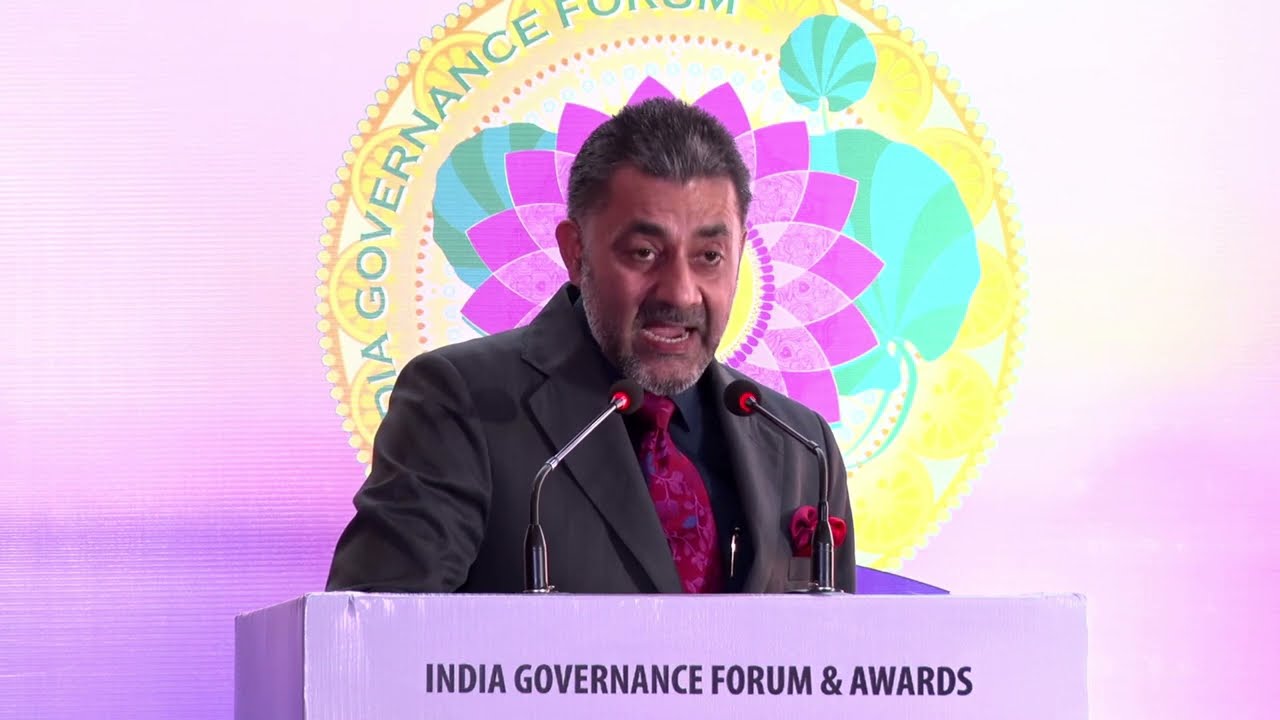This rectangular photograph captures a man speaking at a podium with two microphones. The podium, simple and rectangular, bears the text "India Governance Forum and Awards" in black. The man is dressed in a black suit, black shirt, and a red tie with blue accents. He has short, spiky hair and a neatly trimmed beard and mustache, and his mouth is open as he speaks. The backdrop consists of a projection on a wall shaded in purples, featuring a round seal. This seal showcases a vibrant, multi-colored design with hues of blue, green, purple, pink, and yellow, and prominently displays "India Governance Forum." There is a light source to the right, making that side of the background brighter. The setting suggests he is presenting at an event dedicated to governance in India, with the atmosphere and decorative elements reinforcing the formal and celebratory tone of the occasion.